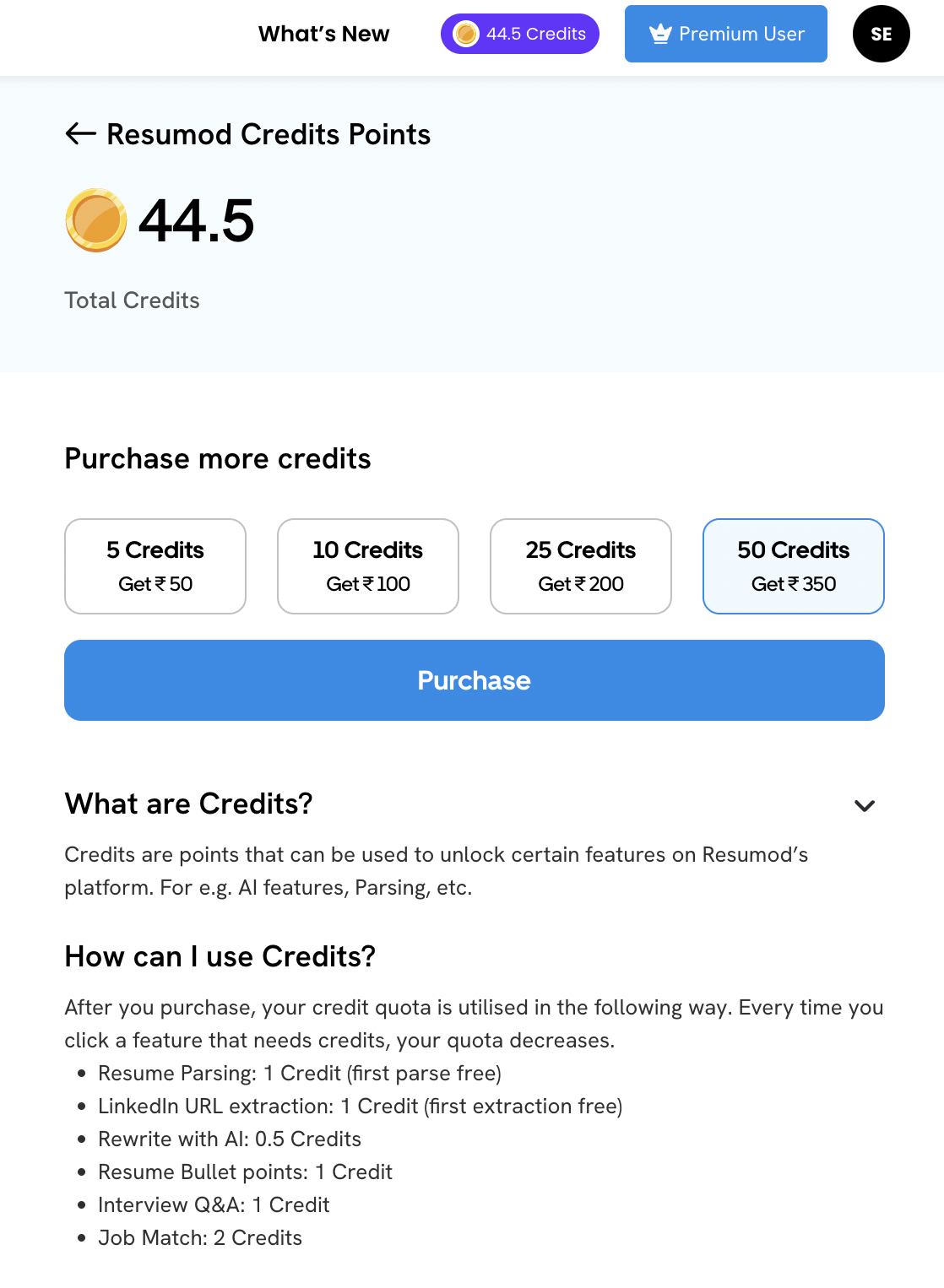In the image, we see a user interface related to a credit system. At the top right corner, there's a black circle with the letters "SE" inside it. Adjacent to this, a white text within a square box indicates "Premium User," accompanied by a white crown icon just to its left. Further left, a purple bubble-shaped box displays "44.5 credits" and is marked with a circle containing a gold coin.

At the top left of the image, the text reads "What's New" in black. Just below this, the text "ResumeMod Credit Points" appears with an arrow pointing left. Next to this text, the number "44.5" is shown beside a gold coin icon.

Centrally positioned in the image, the heading says "Purchase More Credits," followed by four boxes indicating different credit packages: "5 credits," "10 credits," "25 credits," and "50 credits."

Beneath these credit options, there is a blue rectangular box with the word "Purchase."

Further down, two sections provide additional information: one titled "What are Credits?" and the other "How Can I Use Credits?" Both of these sections' titles are in black text.